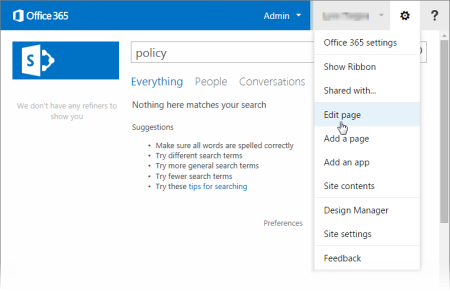This image captures a detailed view of the Office 365 Admin page. Dominating the top of the screen is a bright blue ribbon. On the left side of the ribbon, "Office 365" is prominently displayed in white text, accompanied by the Office logo. To the right, "Admin" is marked with a drop-down arrow next to it. A currently expanded drop-down menu reveals options, with "Office 365 Settings" at the top, followed by "Show Ribbon," "Shared With," "Edit Page," "Add a Page," "Add an App," "Site Contents," "Design Manager," "Site Settings," and "Feedback." The cursor is positioned on "Edit Page," highlighting it in light blue.

Beneath the blue ribbon, there's a search bar where the word "Policy" is entered in gray text. The search options for "Everything," "People," and "Conversations" are shown with "Everything" highlighted in bright blue. Below the search bar, a message indicates no search results with the text: "nothing here matches your search." Suggestions for improving the search, such as making sure all words are spelled correctly, trying different or more general search terms, and using fewer search terms, are listed. The phrase "tips for searching" is highlighted in bright blue, suggesting additional help is available.